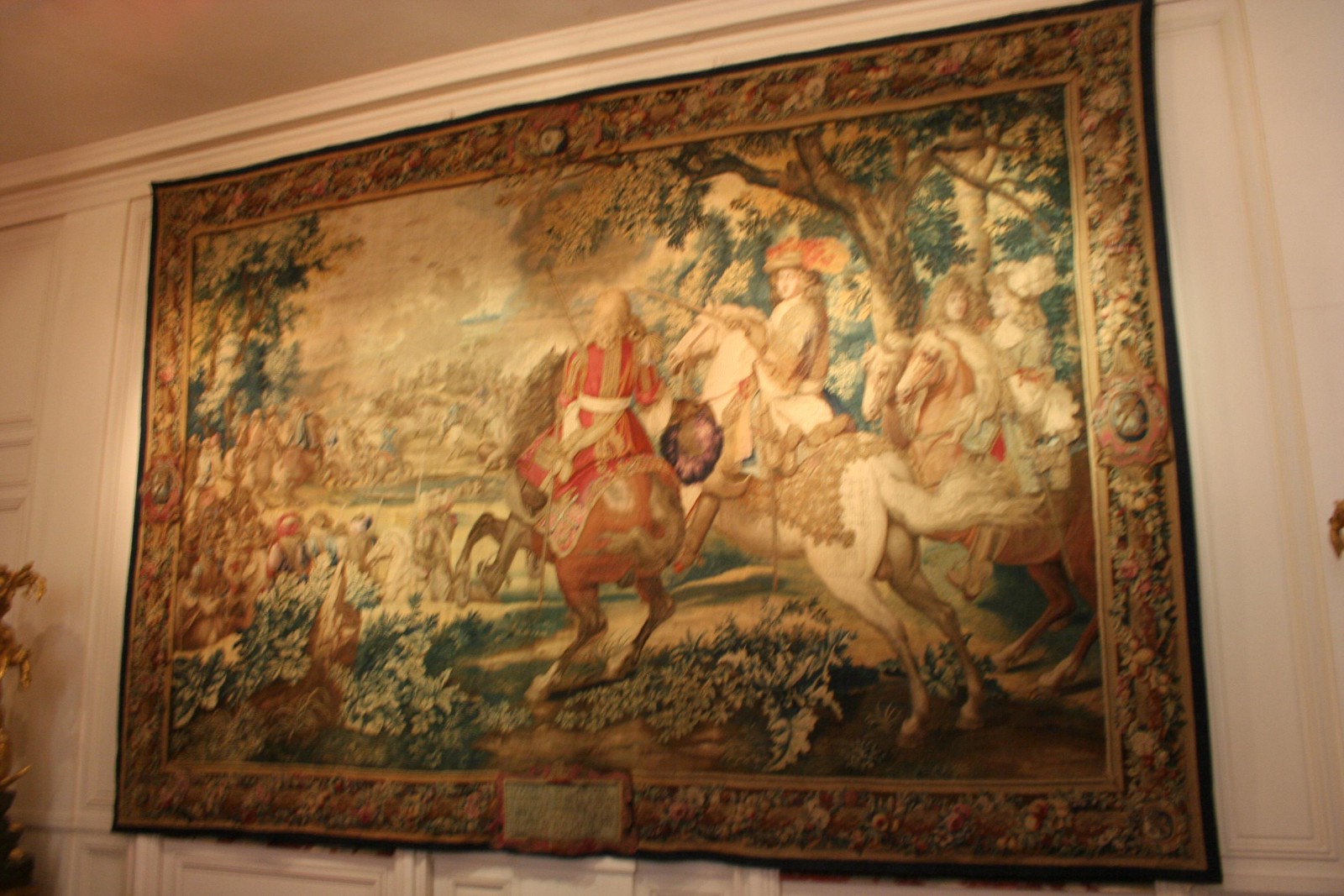This photograph showcases a large, weathered medieval or perhaps Renaissance tapestry, most likely displayed in a smaller museum or a private home. The tapestry is ornately detailed, depicting a scene with four figures on horseback—two in the foreground and two more blurred in the background. The two prominent knights are poised for battle, with one horse white and the other brown, both rearing up dramatically. One knight wears a distinctive, feathered cap reminiscent of French attire. The tapestry is mounted on a white, wood-paneled wall, under neutral lighting that has imparted an orange wash over the scene. The surrounding room features vaulted ceilings with lines of molding, but minimal advanced security or sophisticated mounting, suggesting a more intimate setting rather than a major museum gallery.